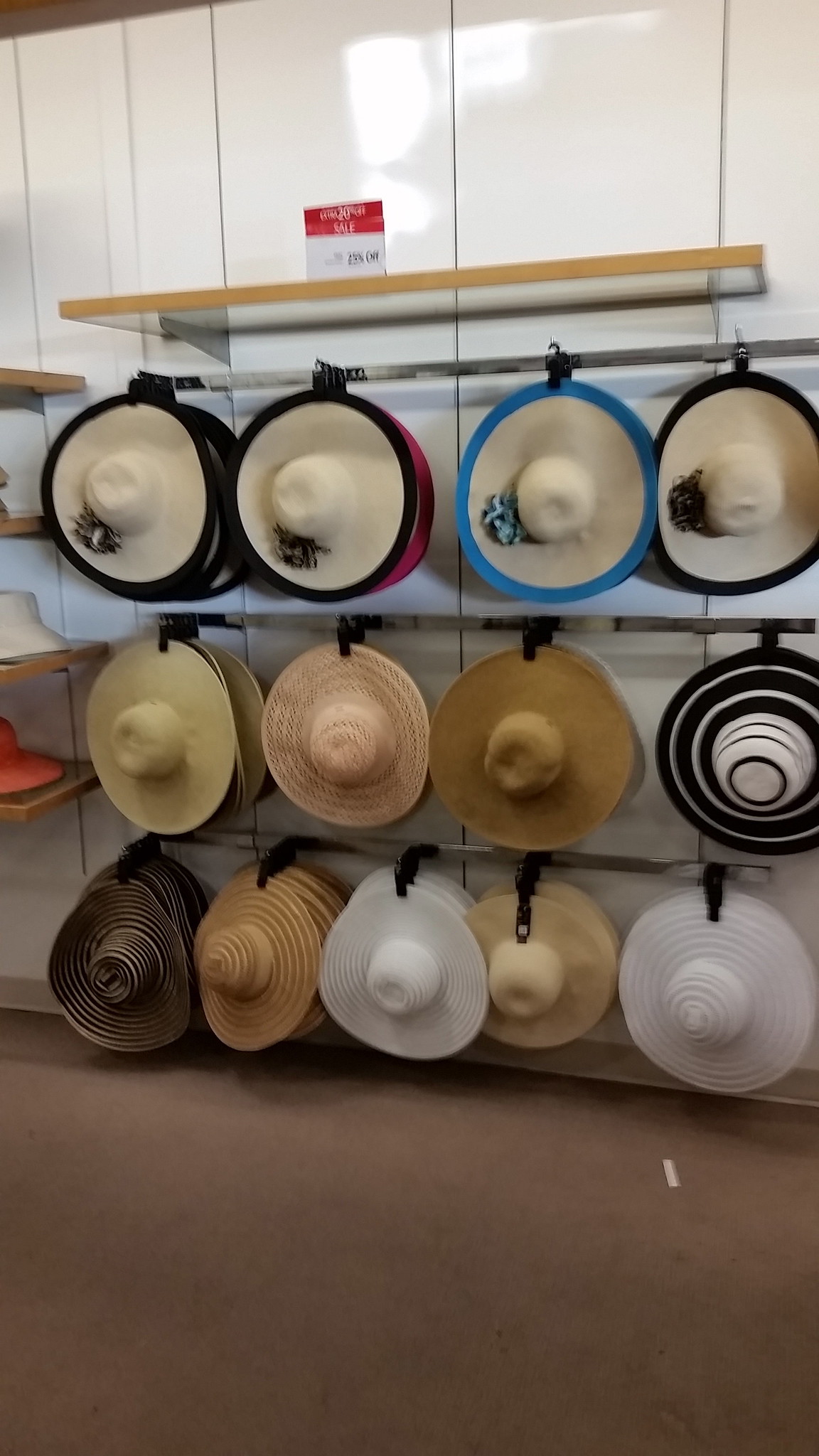The image displays a well-organized display of sun hats and fedoras hanging in a store, presented in three horizontal rows on gray rods. The background features a glossy white paneled wall with a white and red sign above a wood-edged shelf. The hats are made from a straw-like or poly material and are arranged by color and design. The bottom row consists of five fedoras starting with a dark brown hat, followed by a tan one, a white one, another tan hat, and another white hat. The middle row features a tan fedora, a pinkish-brown one, a brown one, and a distinctive black and white circular patterned fedora. The top row displays four hats with black or blue accents: a black and white, black and white, blue and white, and another black and white hat. Below the hats, the floor is covered in brown carpet, and gray baseboards run along the base of the wall. A small section of flat shelves with similar hats can be seen on the left edge of the image.